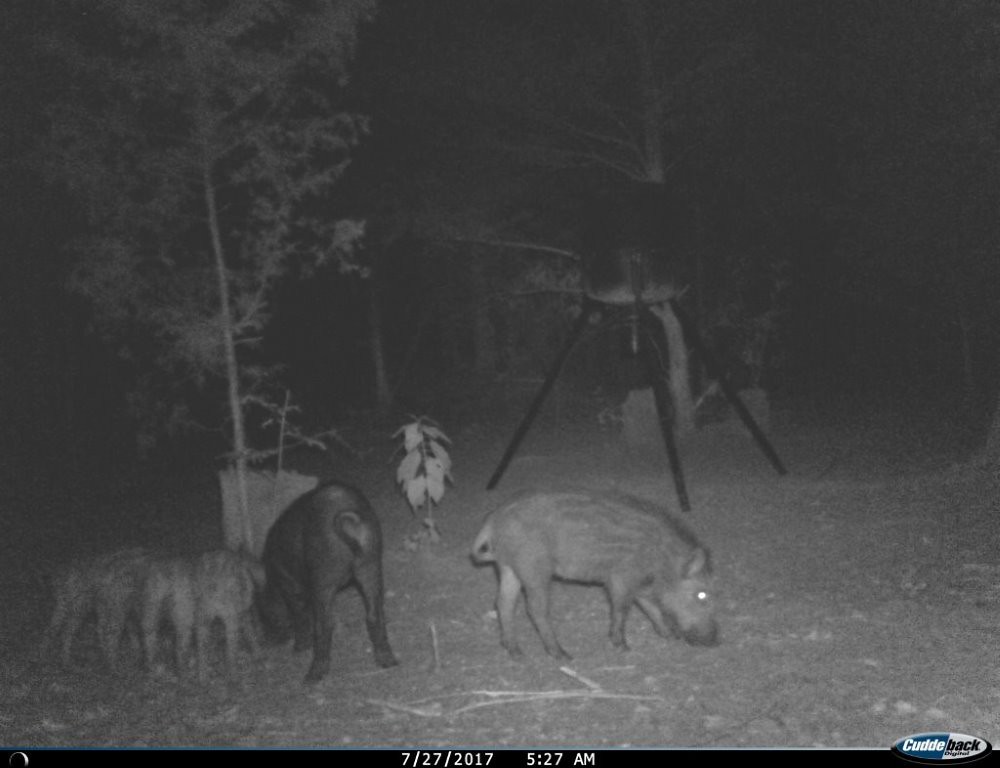This black and white nighttime photograph, captured by a trail camera on July 27, 2017, at 5:27 AM, depicts a woodland scene with several trees scattered around, including thinner trunks and sparse branches. In the foreground, there are six warthogs—their short tails curled at the sides—standing on the dirt ground. The center of the image focuses on a light-colored adult warthog with its head down, seemingly eating something from the ground, one leg extended slightly forward. To its left, a larger, dark-colored warthog is also feeding, with its backside facing the camera and tail curled. Arranged in a semicircle around the dark warthog are four small piglets, lighter in color, also appearing to eat. Visible text at the bottom of the image marks the date '7-27-2017' and time '5.27 AM' in white lettering, and an oval-shaped symbol on the far right that reads 'CUD BACK' in blue and gray. A black camera set up on a tripod can also be seen in the background.